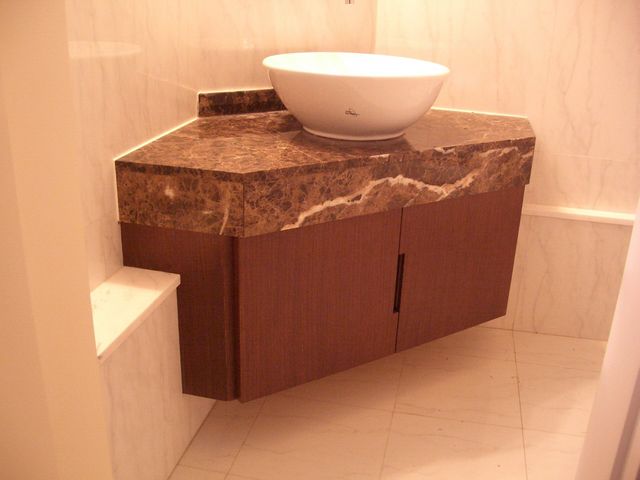This image, whether a photograph or computer-generated, captures a sophisticated and modern bathroom characterized by a blush pink ambiance. The space is enveloped in luxurious marble, with white and gray veins running through the material, evoking a chic and elegant atmosphere. The bathroom features impeccably polished marble tile flooring, matching marble ledges, and walls composed of solid marble slabs.

Taking center stage is an intriguing bathroom cabinet, protruding from the wall at an unconventional angle. The cabinet's countertop is a striking contrast to the room's overall light tones, displaying a darker terracotta-colored marble with intricate white streaks. The expansive sink, which sits fully atop the countertop, adds a bold touch to the design, alongside a minimalist faucet that seemingly descends from above.

The vanity beneath the sink is sleek and minimalist, with flat cabinet doors that forgo traditional handles in favor of built-in handholds. This attention to detail and the unique combination of materials and colors make the bathroom a standout example of modern design infused with classic elegance.